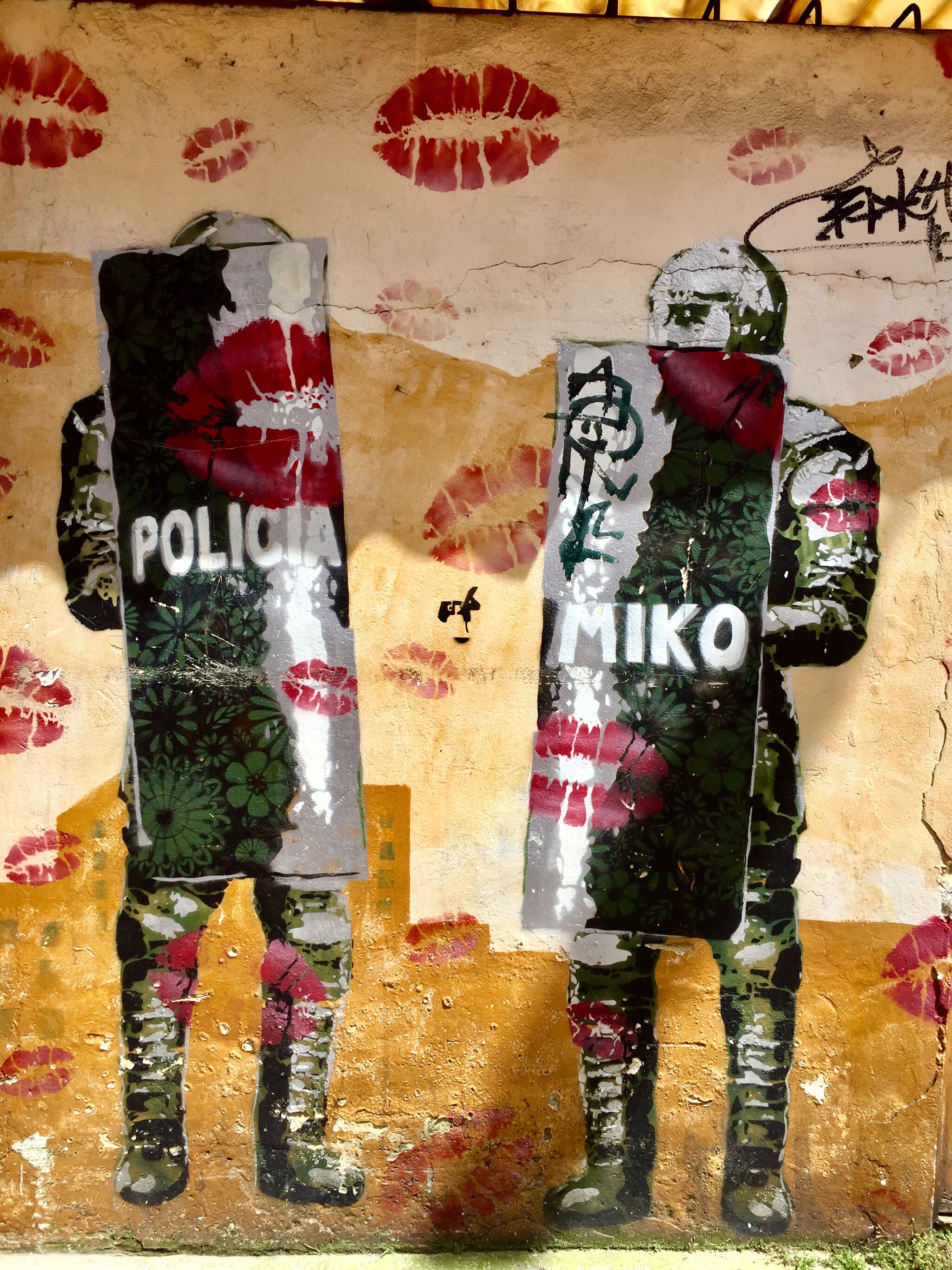The image is a detailed artwork on a hard surface like a stone or cement wall, dominated by graffiti and paintings. At the top of the wall, there's a series of red lip imprints, with a large one centrally placed and smaller, fainter ones to the right. The background displays a gradient of colors: the top third is a light tan color, the middle third is light brown, and the bottom third transitions to an orangey-brown hue. Additionally, some black writing appears on the right side, though it is indiscernible.

Centrally depicted are two figures clad in police gear, complete with fatigues, boots, and helmets. Both hold large police shields bearing distinct markings; the shield on the left reads "POLICIA" and the shield on the right reads "MIKO." Both shields are adorned with red lip prints and green flower designs. The officer on the left is partially obscured by their shield, revealing only the top of their head, a bit of their right arm, and their legs from the knees down. The officer on the right, facing slightly left, has their face partially visible, showing a helmet and part of their left arm, with their left hand concealed behind the shield. Their left leg is visible and the right leg is seen from the knee down.

Surrounding the figures and blending into the overall setting are multiple red kiss marks, detailed enough to show the lines in the lips. The wall's lower edge includes some natural elements like moss or weeds growing up from the ground, adding a touch of realism to the composition. In the corner of the image, there is an artist's signature, marking the creator's identity. Overall, the artwork merges vivid street art elements with a poignant portrayal of law enforcement figures.